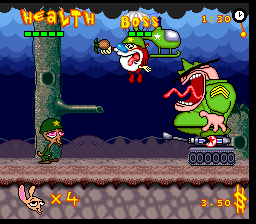This image, seemingly a scene from an old 8-bit video game, features a vivid, hand-drawn, cartoonish design with characters resembling those from 'Ren and Stimpy'. The game area includes both a health and boss bar at the top, each with green squares, the words 'health' and 'boss' highlighted in yellow rimmed with red, and a timer set to 1:30 with a clock icon indicating a timed boss stage.

On the left, a greenish tree stands, adorned with a round, magenta creature who appears to be the main character. This character has an oversized head with a blue nose, large eyes, and is holding what looks like a pineapple grenade. To the right, a caricature of a drill sergeant, complete with a large mouth, green outfit, and yellow-starred helmet, is yelling while standing atop a comically small tank. Below the sergeant, the ground features images of dirt and rocks, adding to the gritty, military aesthetic of the scene.

Hovering in the sky, a green helicopter, detailed with a star symbol, is positioned above the characters with its propellers spinning. On the lower left, the creature has "x4" next to it, indicating four lives, while the lower right corner displays a dollar sign followed by "3.50", suggesting the player's in-game currency. Overall, the detailed combination of elements captures a whimsical yet intense boss fight in a nostalgically styled video game.